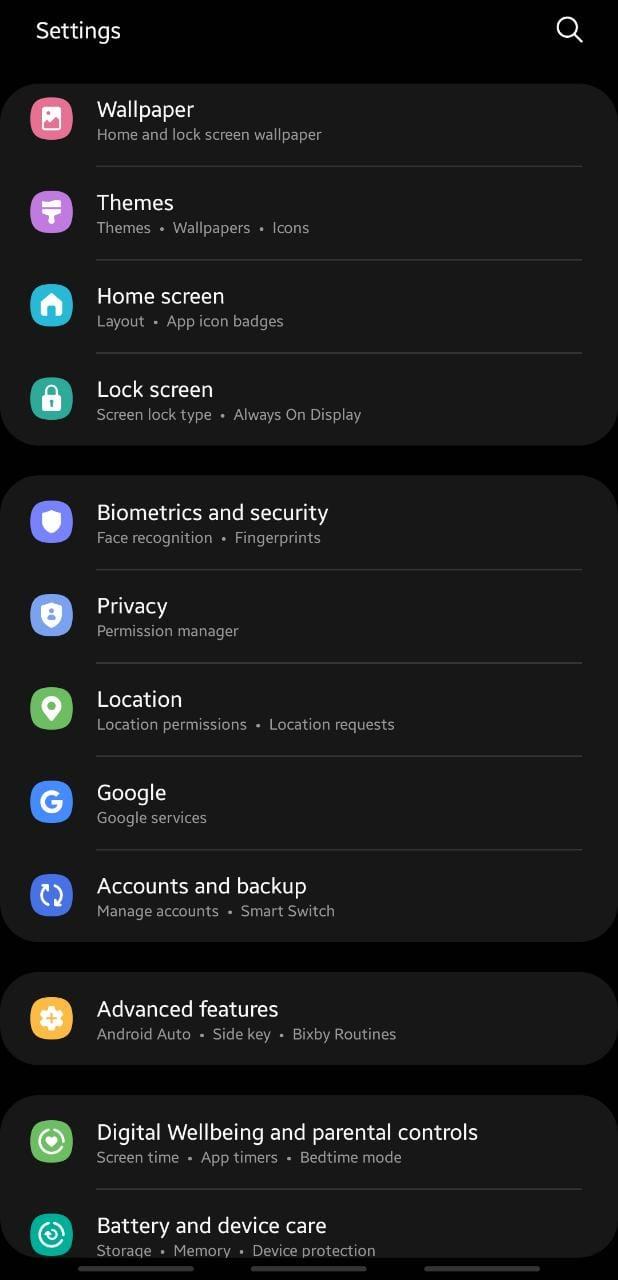This screenshot displays the settings menu of a device with a sleek black background and grayish-white text. The top of the menu features a "Settings" header alongside a magnifying glass icon, indicating a search function. Below that, the menu items are organized with clear labels and corresponding icons.

1. **Wallpaper**: A section with a pink icon featuring a white box, labeled "Wallpaper," where users can customize both home and lock screen wallpapers.
2. **Themes**: This section, marked by a purple icon with a white paintbrush, is labeled "Themes," and provides access to themes, wallpapers, and icons.
3. **Home Screen**: Identified by a light blue icon with a house image, this section is labeled "Home Screen" and allows users to adjust the layout and app icon badges.
4. **Lock Screen**: This section has a greenish-teal icon with a padlock and is labeled "Lock Screen," offering options for screen lock type and Always On Display.
5. **Biometrics and Security**: With a blue icon featuring a shield, this section is labeled "Biometrics and Security," providing settings for face recognition and fingerprints.
6. **Privacy**: A light blue icon with a shield and person marks this section, labeled "Privacy," which includes a permission manager.
7. **Location**: Identified by a green icon with a white location pin, this section labeled "Location," provides settings for location permissions and location requests.
8. **Google**: This section has a blue icon with a white "G," labeled "Google," and includes settings for Google services.
9. **Accounts and Backup**: A blue icon with white arrows marks this section labeled "Accounts and Backup," offering options for managing accounts and using Smart Switch.
10. **Advanced Features**: An orange box with a white cogwheel icon identifies this section, labeled "Advanced Features," which includes settings for Android Auto, side key functions, and Bixby routines.
11. **Digital Well-being and Parental Controls**: Labeled "Digital Well-being and Parental Controls," this section, with a green box and a white circle and heart icon, covers screen time, app timers, and bedtime mode.
12. **Battery and Device Care**: Featuring a teal icon with a white circle, this section is labeled "Battery and Device Care," and includes settings for storage, memory, and device protection.

At the bottom of the menu, there are three gray dashed lines, likely indicating additional menu items or a scroll bar.